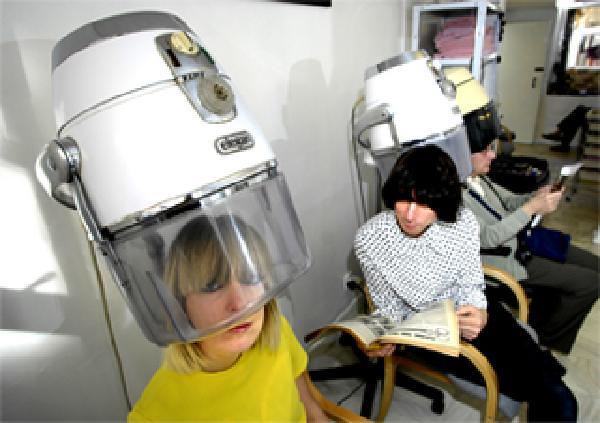The photo captures a modest beauty salon with a linoleum floor and a row of vintage hair dryers along the left wall. In the foreground, a woman wearing a bright yellow T-shirt sits under one of these old-fashioned head dryers, staring directly at the camera with heavily lined eyes and shoulder-length blonde hair that loosely falls into her face. Her hair appears dry, raising questions about why she's under the dryer. Behind her, two other customers also sit under the dryers; one is a man with long, nearly shoulder-length hair obscuring his face, engrossed in a magazine. The second is a person just barely visible, also reading a magazine. The salon appears to lack stylists in the scene, and the decor includes a white door in the top right corner and possibly a supply shelf or bookcase. The overall feel, accentuated by the customers' outfits and the evident digital compression of the photo, suggests it’s from an era like the 90s. The image captures a quiet, routine moment in this timeworn salon.